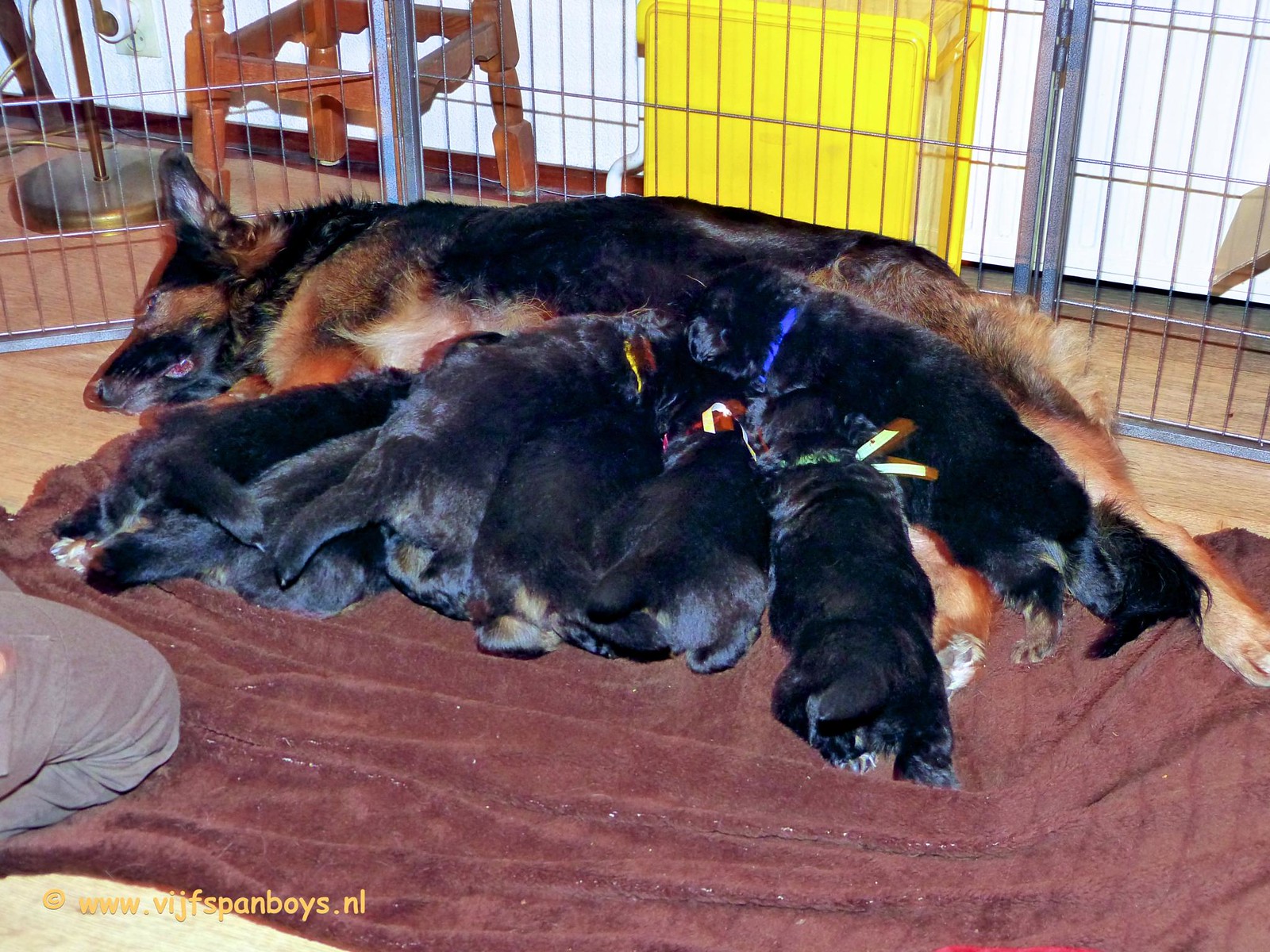The photograph, likely sourced from the website www.vijfspanboys.nl, captures an intimate scene of a mother German Shepherd, or a dog resembling one, nursing her large litter of puppies. The image, taken from an overhead perspective, showcases the puppies—distinctively black and clearly past their newborn stage—arranged in a row and nursing from their mother who is reclining on a fuzzy brown blanket. The setting includes a gated pen made from interconnected panels, situated on a brown wooden floor. Outside the pen, there's a white wall, a yellow object, and the bottom section of a brown wooden stool or perhaps a lamp base. An unidentified gray object and a pair of legs in gray pants, possibly belonging to a person kneeling nearby, are also visible. This cozy scene unfolds in front of a silver metal cage barrier. The overall vintage appearance of the room suggests this image might not be from a very recent period.